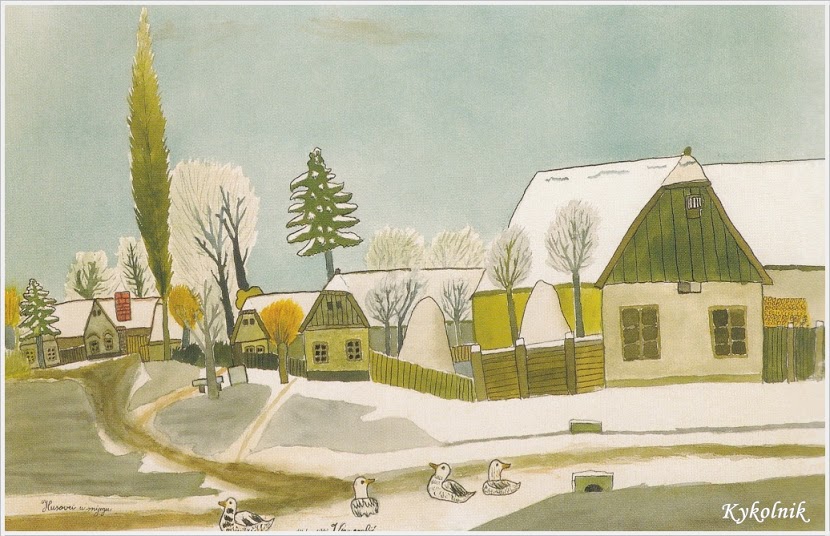This painting by the artist Kai Kolnick, whose name is signed in the lower right corner, depicts a charming winter scene by a series of cottages. The colors are primarily light blue, lime green, yellow, brown, and off-white. The sky has a light winter blue hue, adding to the serene atmosphere. The foreground features four ducks, either floating or sitting by a frozen or partially frozen stream. The ground around the ducks has a mix of snow-covered areas and clearer patches.

The middle ground showcases five quaint, one-story cottages, each with slightly wobbly yet straight-lined A-frame roofs topped with snow. The cottages are painted in shades of green and yellow, with vertical wooden slats extending from the roof to the base. Wooden fences of varying shades connect the cottages, along with a few details like benches and brick chimneys.

Scattered trees add to the wintery feel; most are barren of leaves except for a towering fir tree in the left center, which retains its needles and rises into the sky. The snow-laden rooftops and the varied green hues of the cottages contribute to a rustic, appealing ambiance, making the painting a captivating portrayal of a tranquil winter's day.